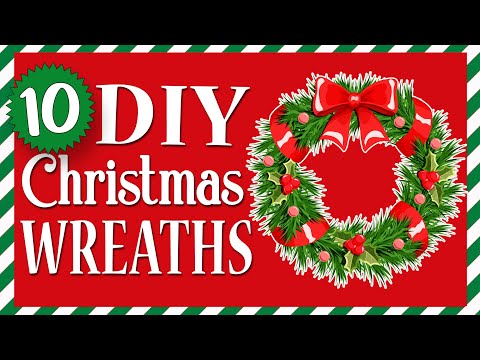The image depicts an illustrated Christmas card against a black background. The rectangular card features a border with green and white diagonal stripes. Inside the border, the card has a bold red background. On the top left side, there is a green circular emblem with a pointy edge containing the number "10." Below this emblem, in all-capital white letters, the text reads "DIY Christmas Wreaths." On the right side of the card, there is a detailed illustration of a Christmas wreath made of green holly leaves. The wreath is adorned with a red bow at the center top, and a red ribbon is elegantly wrapped around it. Scattered around the wreath are red circular ornaments and red hearts, capturing the festive spirit of old Christmas traditions.